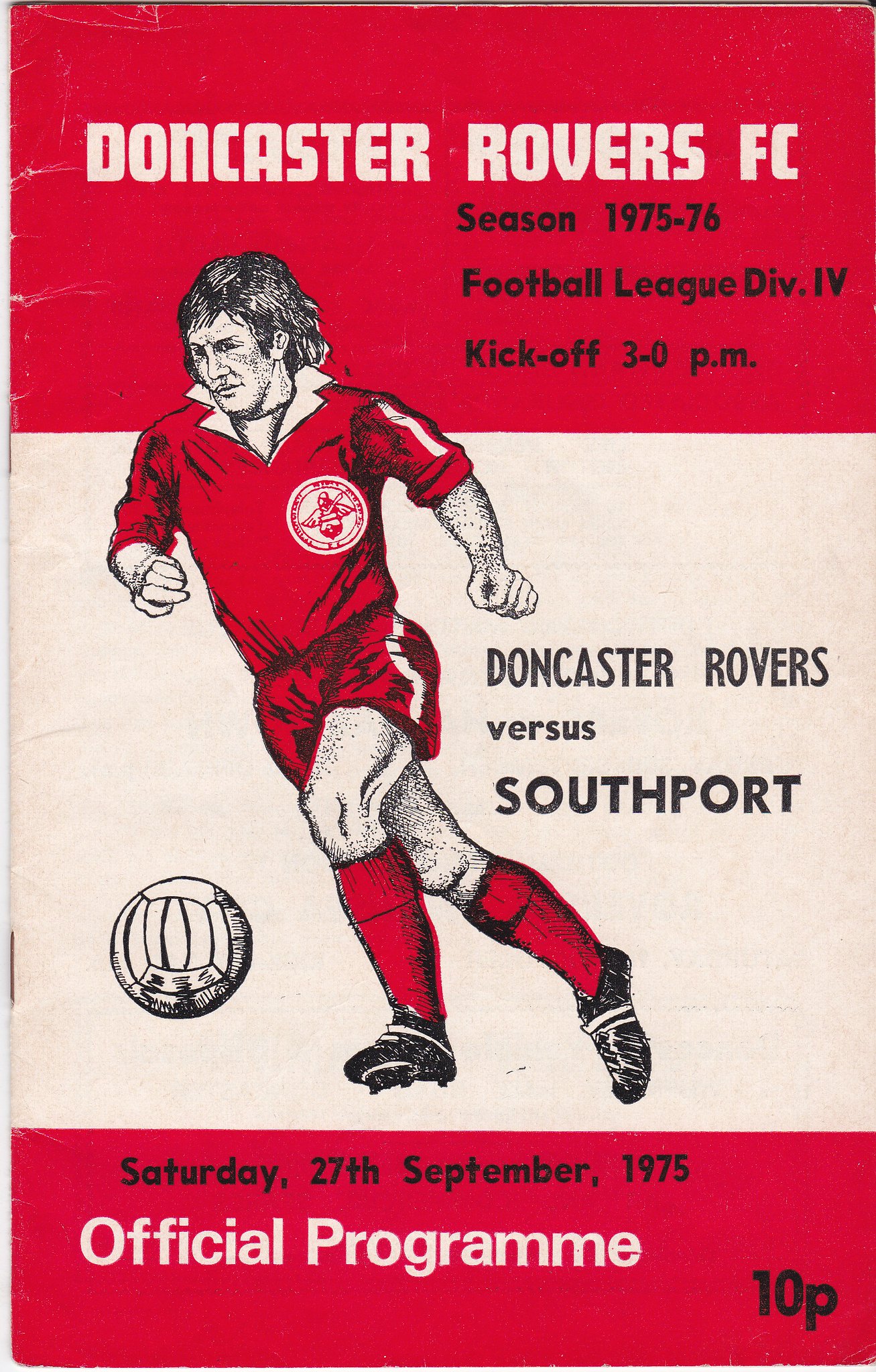The image is the cover of an official game program for a soccer (or football) match between Doncaster Rovers and Southport, dating back to the 1975-76 season. The background of the program is primarily aged white, giving it a pinkish hue. The top and bottom of the cover feature red banners. The top quarter of the page is dominated by a red rectangle with "Doncaster Rovers FC" written in white. Below this, black text reads "Season 1975-76 Football League Division IV" with the number four in Roman numerals (IV), followed by "Kickoff 3-0 p.m." The center of the cover showcases a hand-drawn image of a male footballer in a red uniform, complete with detailed club emblem on the left breast, red shorts with white stripes, and black football shoes. The player is depicted in action, running to the left and about to kick a soccer ball with his left foot. Flanking this illustration, also in black text, are the words "Doncaster Rovers versus Southport." The bottom red banner has the date "Saturday, 27 September 1975" in black and the words "Official Program" (with the British spelling "Programme") in white. In the bottom right corner, the price is marked as "10p" or 10 pence. The cover also shows signs of age, such as creases and visible staples along the spine.